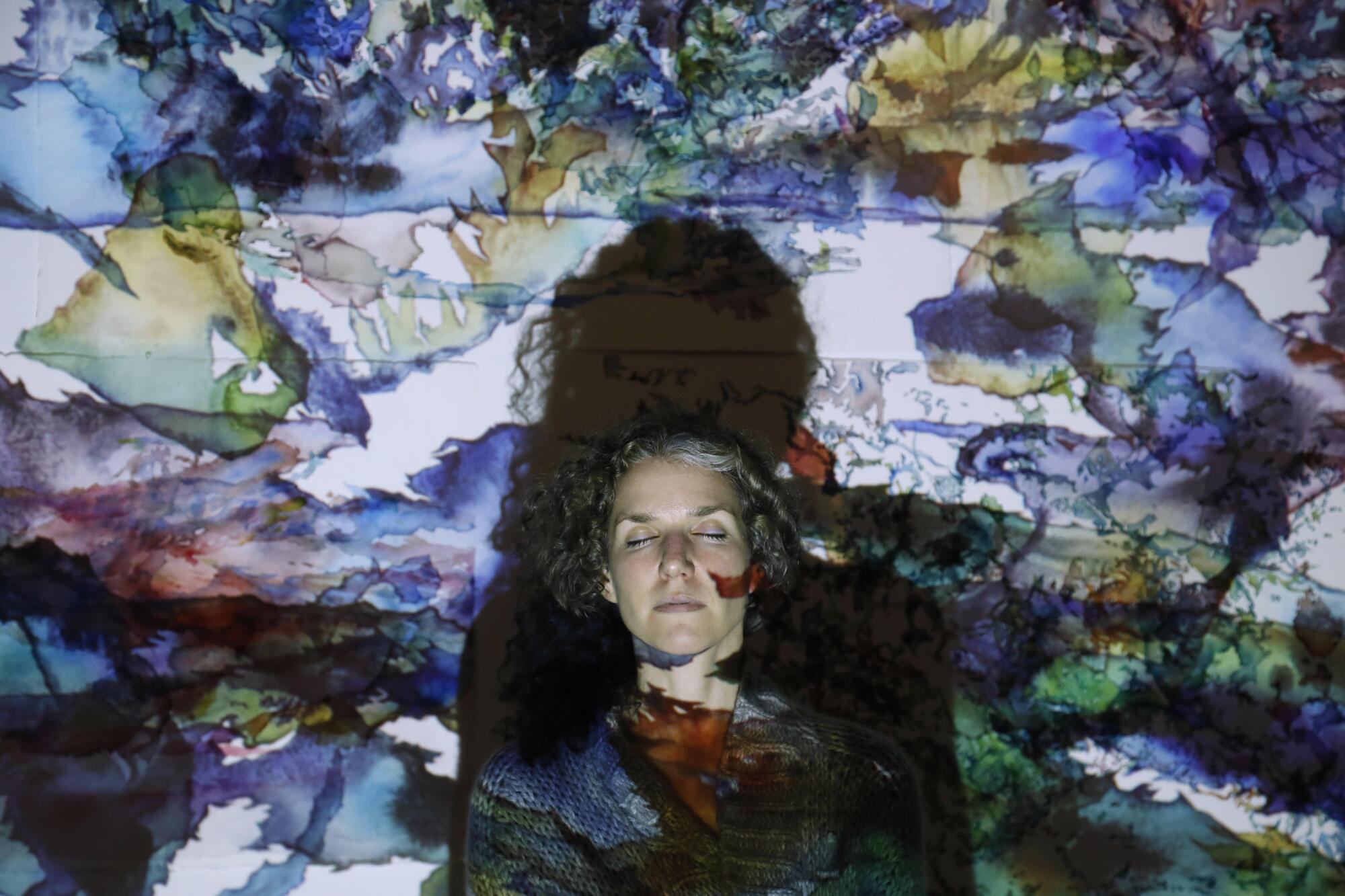In this artistic and evocative horizontal photograph, a woman, seemingly in her 40s, serves as the central focus. She stands in front of an inky, shadowy background filled with abstract shapes and patterns rendered in a palette of blues, greens, purples, yellows, and sporadic touches of pink and white, resembling either stained glass or bleeding ink. The setting has a dark, atmospheric feel, potentially shot at night or in a dimly lit room. The woman, with closed eyes and lips, exudes a sense of calm or introspection. She has short, curly hair with hints of gray, particularly on the top right side, and is wearing a dark-colored textured knit top or jacket that melds seamlessly with the hues around her. Her figure casts a large, distinct shadow behind her, creating a striking silhouette that almost appears as an open doorway within the sea of colors. This interplay of light and shadow, coupled with the abstract background, forms an enigmatic and visually compelling scene.